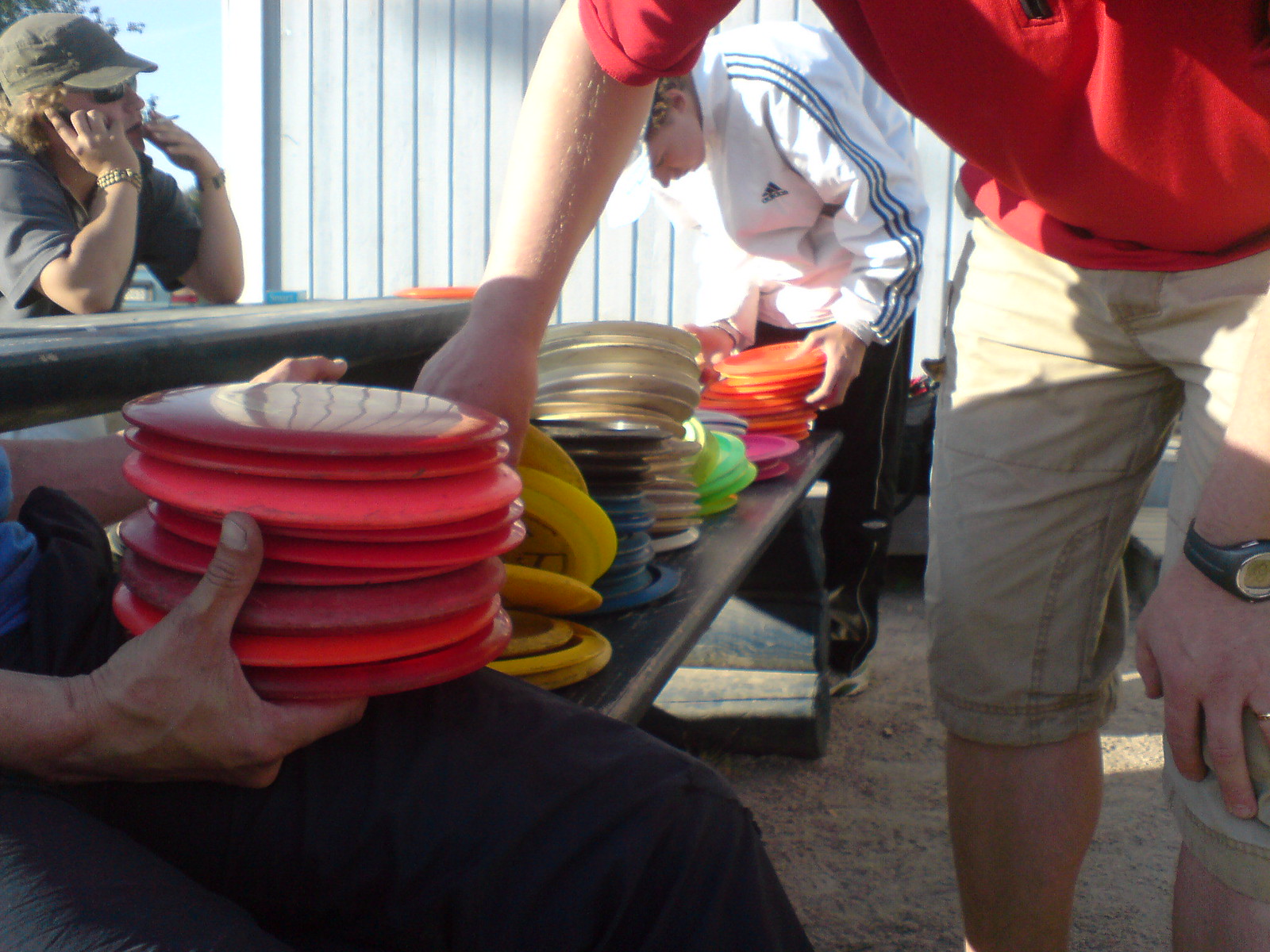In this outdoor image, a diverse array of colorful plates and bowls is stacked on a black wooden table. In the foreground, a person sitting at the edge of the table holds up a vibrant stack on their lap with both hands. Other individuals are closely examining the assorted dishes, contributing to a bustling scene. To the right, several people bend over the table, engaged in sorting through the variously colored stacks. A person clad in a white Adidas jacket with blue stripes is visible in the background, reaching for a set of orange plates.

On the left side of the image, a person wearing a gray shirt, green hat or sunglasses, and accessorized with red and gold wristbands is seated at another table. This individual appears to be smoking a cigarette and talking on the phone. The setting is covered in sand, lending a casual, seaside atmosphere to the scene. In the background, a clear sky and a shed-like building complete the relaxed, outdoor environment.